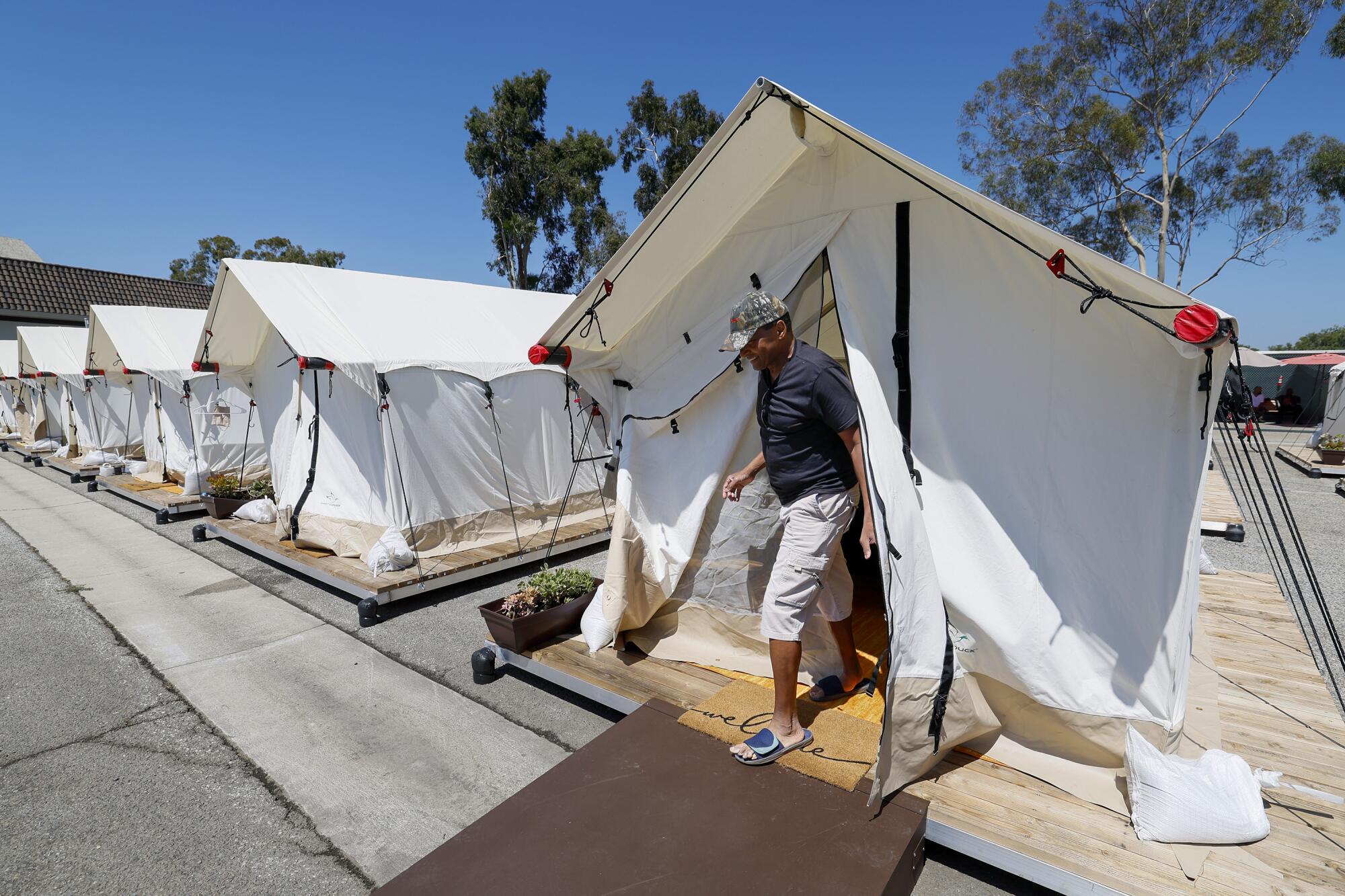This photograph captures a meticulously organized campsite with a series of five neat, identical white tents, each erected on its own wooden platform. The platforms rest on a large concrete slab that appears to be part of a parking lot or other paved area. The row of tents extends from the foreground in the right center back all the way to the left edge of the photo. The sky overhead is bright blue and cloudless, with a few sparse trees visible in the background adding a touch of greenery to the scene. In the foreground, one tent features a man emerging from it, wearing a blue and white baseball cap, gray t-shirt, long shorts, and slide-style sandals. A brown welcome mat lies at the entrance of his tent. The serene weather and the man's apparent smile suggest a pleasant day, adding to the overall inviting and well-ordered atmosphere of the campsite.